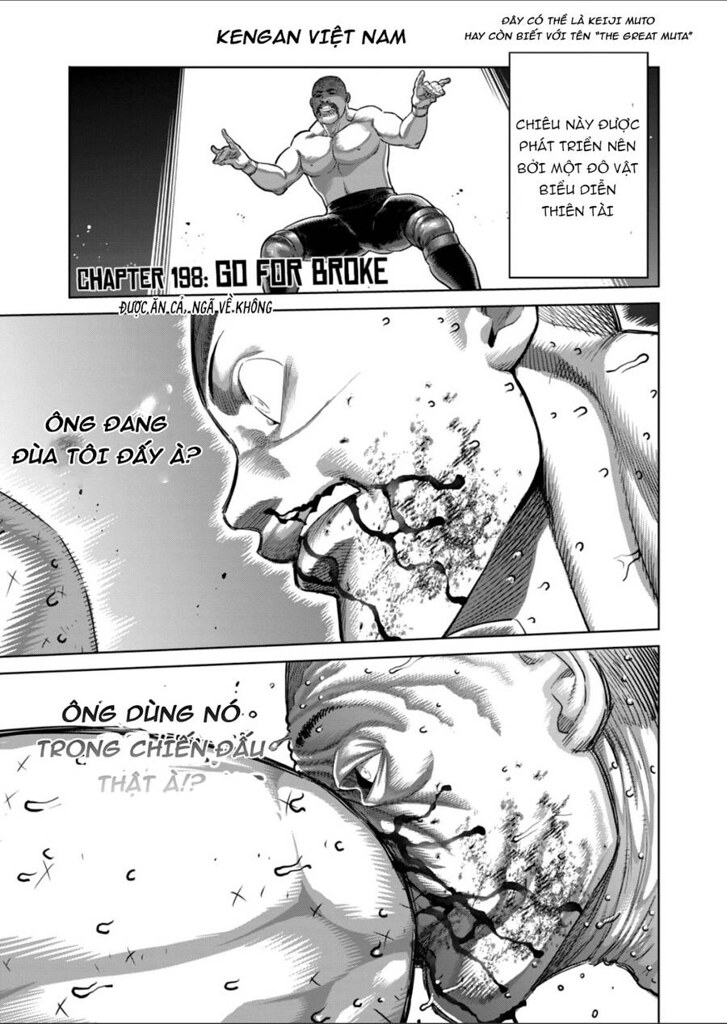This image is a black-and-white comic strip composed of three panels, stacked from top to bottom, and appears to be in Vietnamese, featuring "Kangen, Vietnam, Chapter 198: Go for Broke." In the first panel, a large, muscular man with a bald head and a prominent mustache is shown wearing tight black pants. He is kneeling or squatting with his hands raised, making a devil sign. The second panel provides an up-close view of a different man's face, which is heavily bloodied, with blood streaming from his nose and covering his lips and mouth. The final panel depicts a dramatic action scene where an elbow smashes into this man's face, further smearing blood across his features. The comic's black-and-white aesthetic, drawn with pen or pencil, adds to the intensity and drama of the depicted scenes.